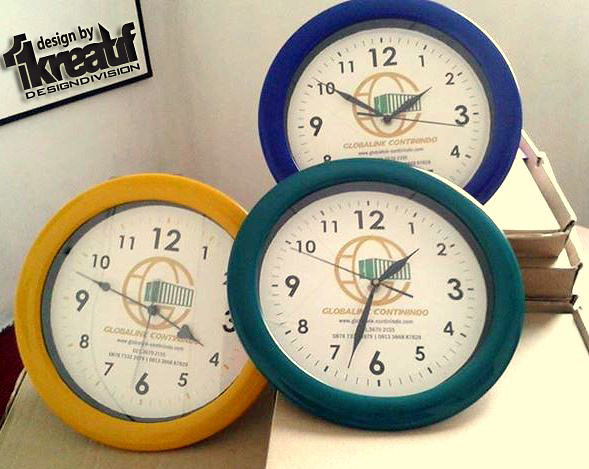This indoor daytime photograph captures a distinctive arrangement of three clocks on a desk, forming an L-shape layout. The top clock features a blue trim and is partially obscured by the clock below it, which has a teal rim. Positioned to the bottom left is a clock with a yellow border. Each clock displays a white face with black numbers and minute markers, centering around a logo of a gold circle intersected by a blue line. The top clock shows a time of approximately 1:33, the teal clock at the bottom reads around 1:33, and the yellow clock displays 3:47. Nestled under the top clock are two cardboard boxes, likely containing paper. To the left of the clock arrangement, a sign on the wall reads "Designed by 1KREATIF, Design Division," outlined in black.